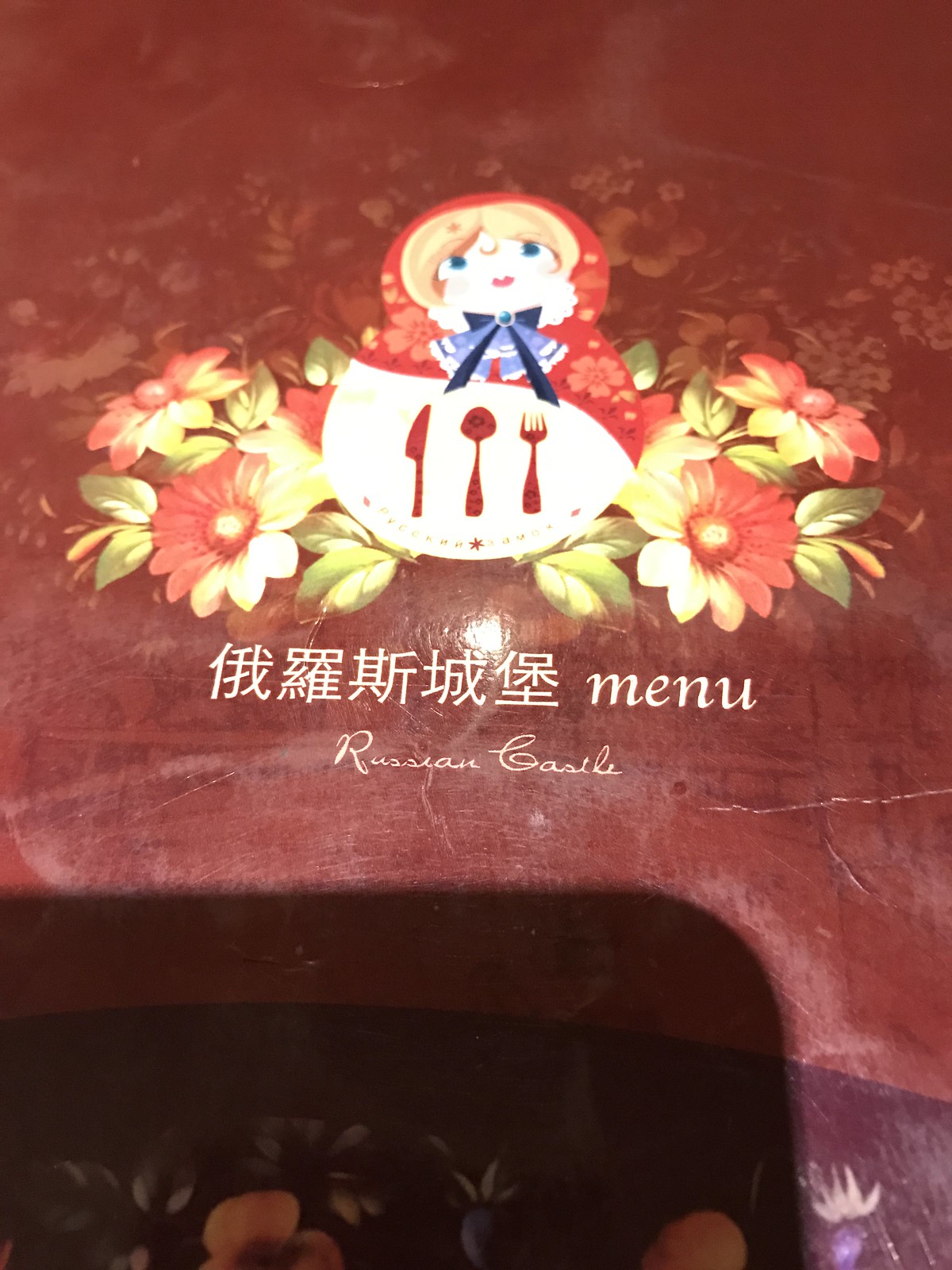The photograph depicts a menu with a reddish-maroon background. In the bottom left-hand corner, a large rectangular shadow—presumably cast by the phone used to take the picture—stretches toward the bottom middle of the image. At the top center of the menu, there is an illustration of a young girl with striking blonde hair, blue eyes, and a heart-shaped mouth. She wears a red hood and a light blue shirt, accented with a white border and a blue bow just below her chin. A white area beneath the bow features a red-colored knife, spoon, and fork. Flanking this central illustration are two flowers on either side, each a blend of reddish-yellow hue with green leaves. Beneath the artwork, written in intricate characters, possibly Chinese or Japanese, is the word "menu." Further below, in English, the text reads "Russian Castle."